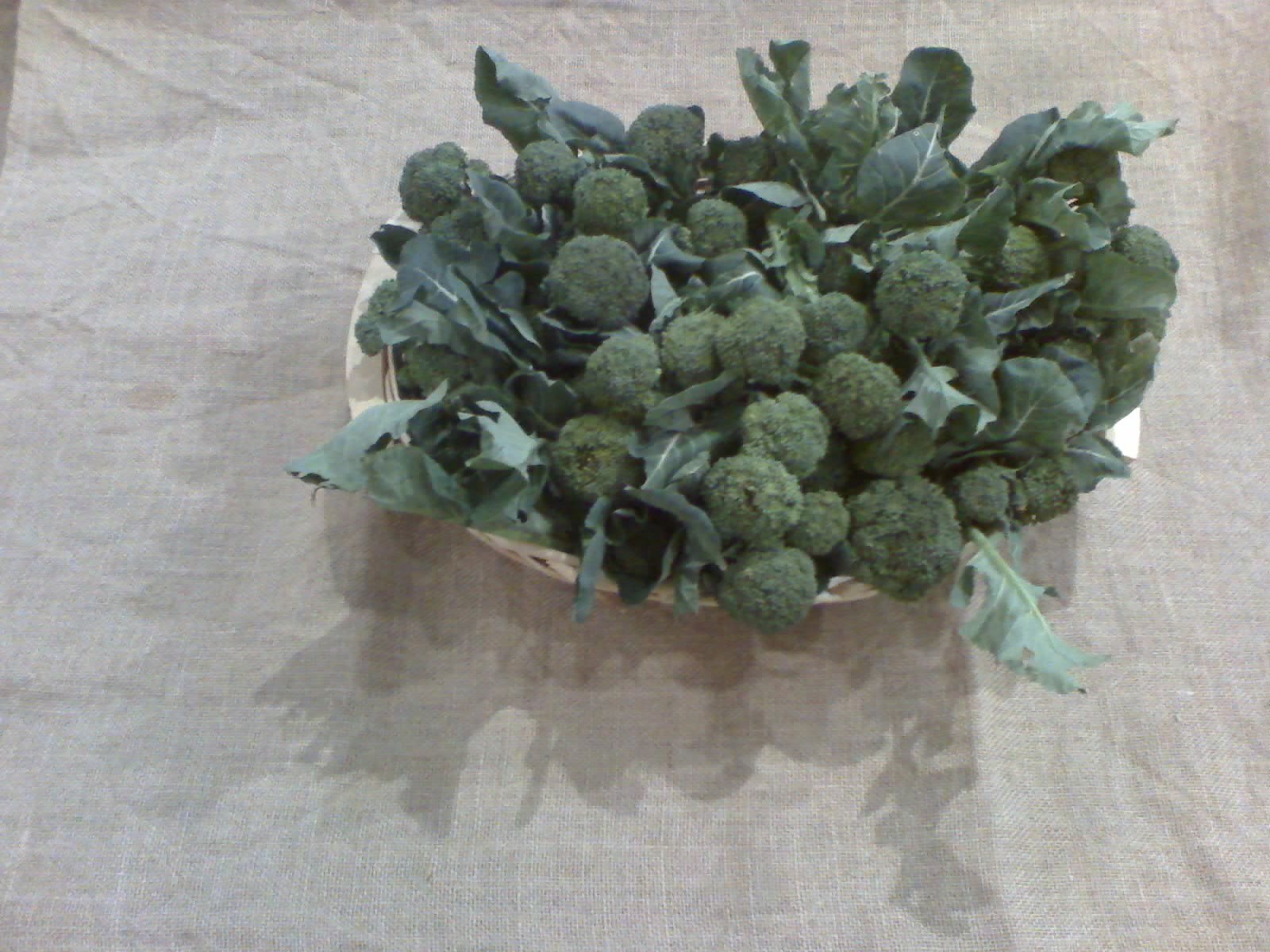The color photograph features a close-up view of a bountiful harvest, placed against a backdrop of a light-colored cloth, likely a beige tablecloth exhibiting several folds, particularly noticeable in the upper left corner. At the center of the image is a white bowl partially visible around the edges and beneath the vegetable. The bowl is filled with what appears to be a type of broccoli, characterized by small, dark green florets and long, thin, dark leaves. The vibrant, healthy-looking vegetables cast a prominent shadow in front of the bowl, adding depth to the scene. The texture and ripples of the cloth beneath enhance the natural, rustic appeal of the photograph.